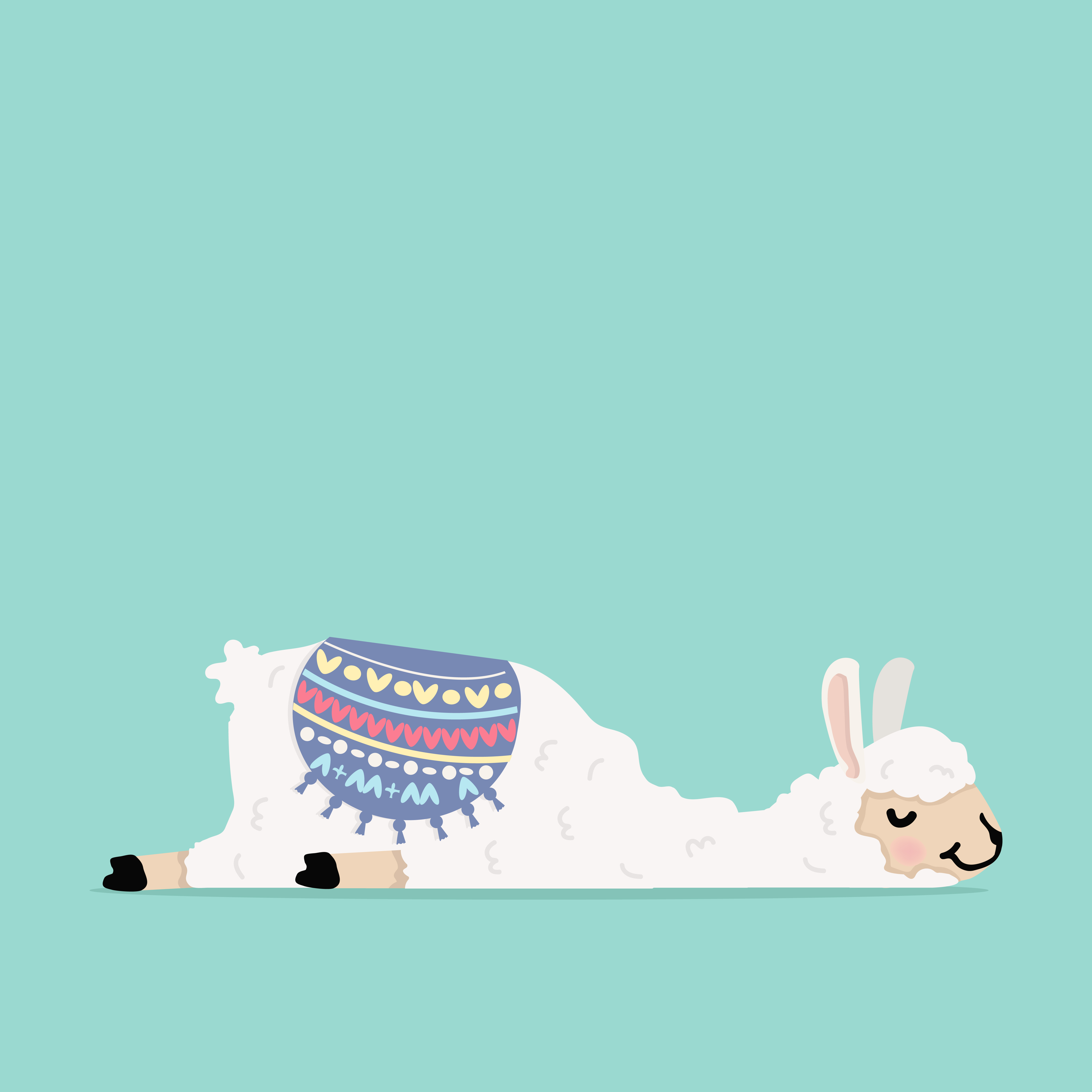In this vibrant, square painting with a teal background, a cartoonish sheep is depicted laying flat on its belly, its legs fully outstretched behind it. The sheep's eyes are closed, and a smile graces its face, enhanced by a pink, rouge-like dot on its cheek. Its unusually long, bunny-like ears, pointed straight up, have a pink inner lining. The sheep boasts a fluffy white body with pink legs and black hooves. Draped over its back is a blue saddle blanket adorned with tassels, featuring intricate designs: yellow hearts and circles, red squiggly lines, white dots and dashes, as well as letter A's and pluses. The charming simplicity of the illustration evokes the style of a children's book, with a clear focus on the whimsical and cheerful depiction of the sheep in repose.